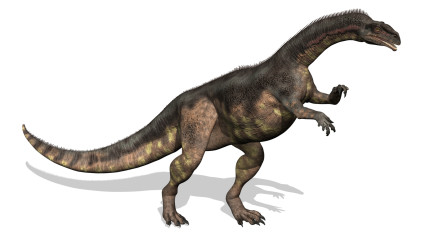This image features a digitally created dinosaur, resembling a hybrid between a Tyrannosaurus rex and a long-necked species. The dinosaur is depicted in a dynamic, fighting stance on its powerful hind legs, facing the right side of the frame, with no background to anchor it. The creature is adorned with gray, leathery skin and detailed scales. A prominent feature is its long, muscular tail that extends in an arced pattern towards the left side. The back leg muscles are visibly strong and robust, supporting its upright posture. The dinosaur's neck is notably longer than that of a typical T-Rex, with small spikes running along the top, leading to a small, lizard-like head. Its short front arms are extended upwards, enhancing its fierce appearance. A shadow cast below the model suggests depth and realism, complementing its detailed and meticulous design.